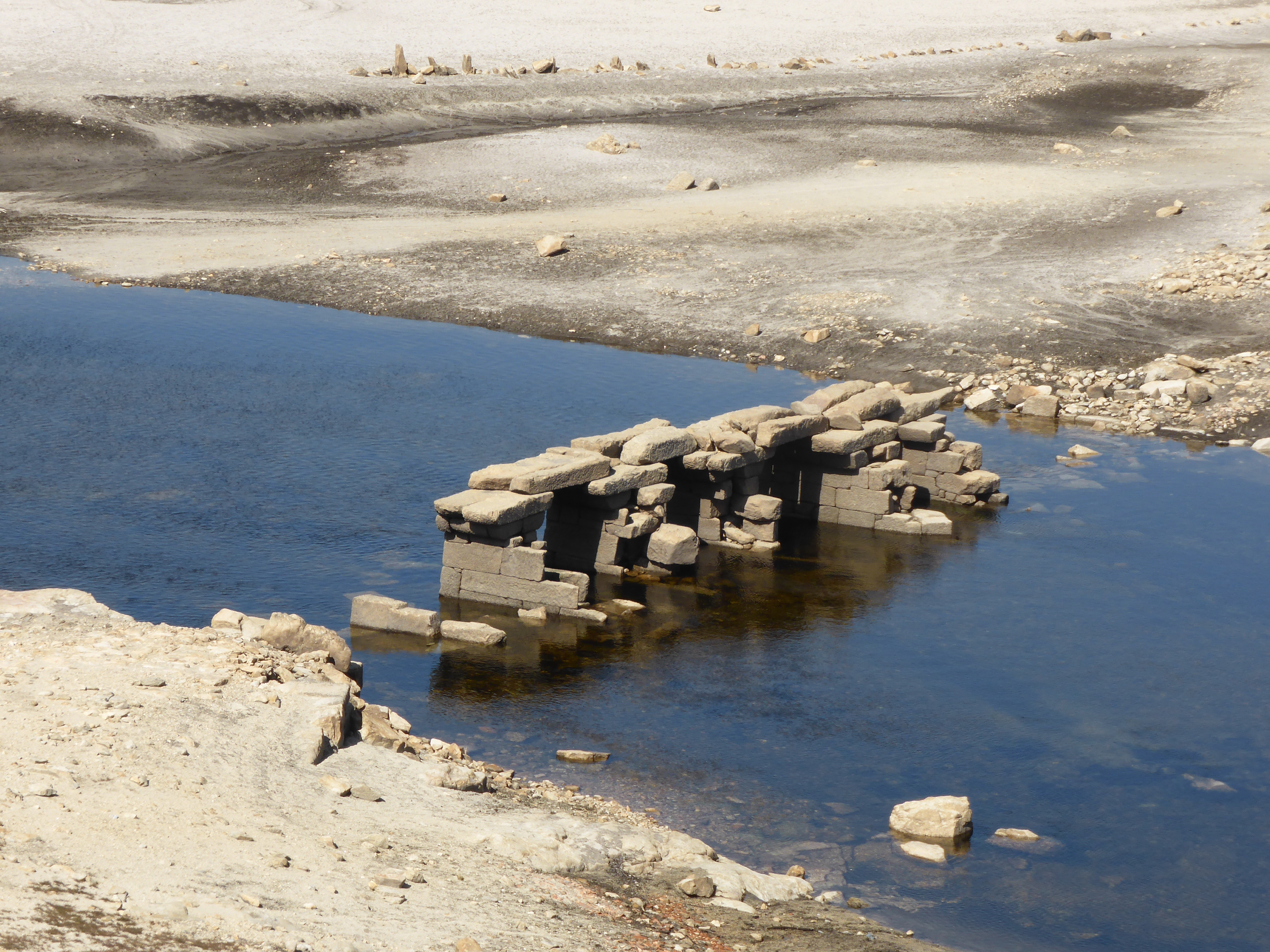The photograph captures a desolate, arid landscape dominated by a large, murky body of water that appears to be a lake, creek, or stream. The central focus of the image is the remnants of an old bridge that once spanned the breadth of the waterway. The bridge has clearly collapsed, with only its base structures remaining, formed from cement blocks and stacked rocks. The ruins extend into the murky dark gray water, where additional debris from the bridge, including fragments of blocks and rocks, can be seen partially submerged. The banks on either side of the water are composed of whitish clay or sand, starkly barren with no visible vegetation, emphasizing the dry nature of the surrounding environment. The overall scene suggests a once-functional crossing now lost to nature's inexorable forces.